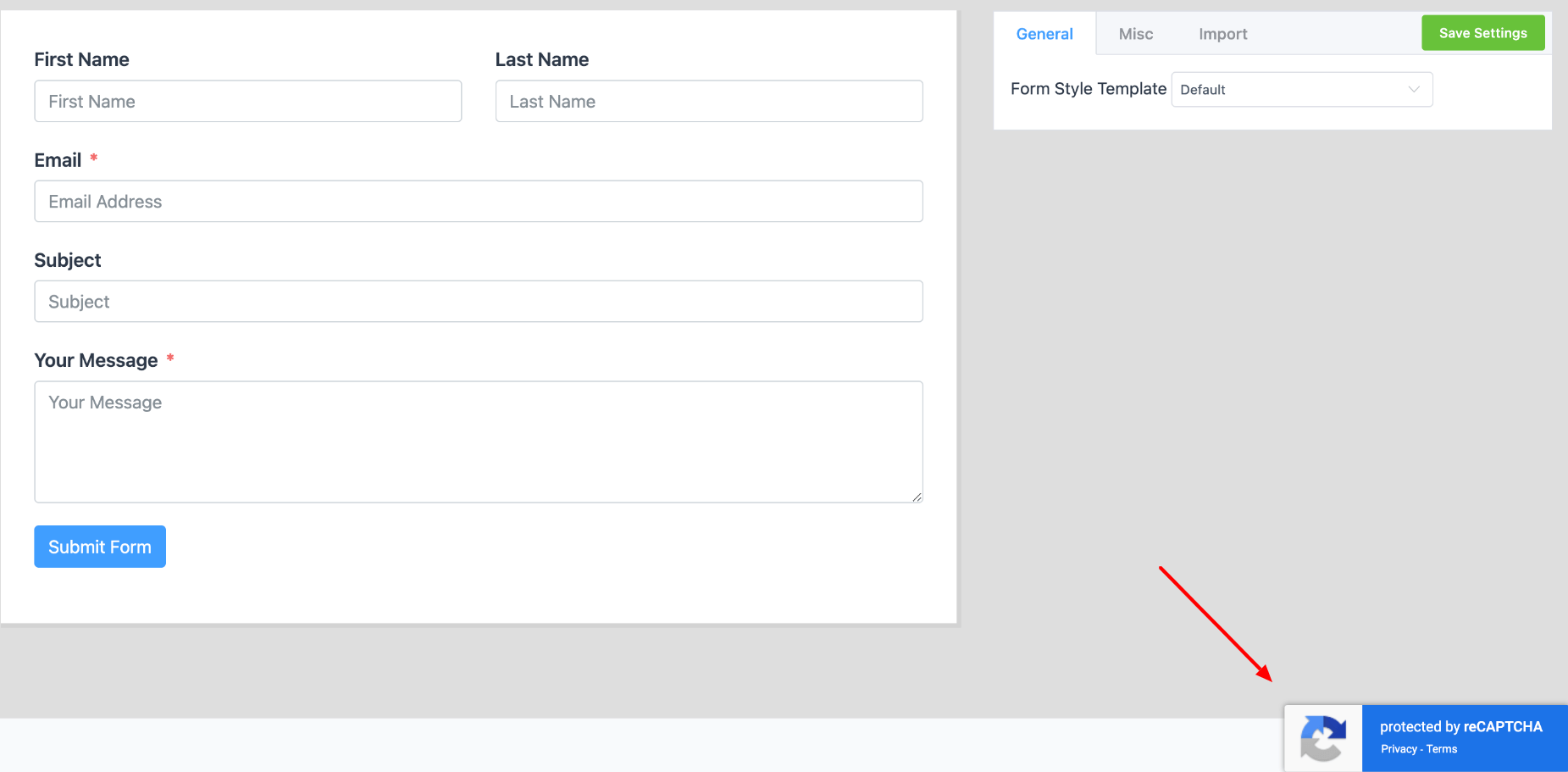In this image, we see a detailed screenshot of an online form interface designed for user input. On the left side of the screenshot, there is a prominent rectangular section featuring a series of labeled text boxes intended for user data entry. At the top, there are fields for "First Name" and "Last Name." Directly below these, a text box is labeled "Email" for entering an email address. Further down, another text box is labeled "Subject," and at the bottom of this section is the largest text box labeled "Your Message" for users to input their message content. 

Situated at the lower left corner of this rectangle is a blue button with white text that reads "Submit Form."

On the right side of the screenshot is a smaller rectangular section with three clickable tabs positioned in the upper left corner, labeled "General," "Miscellaneous," and "Import." Currently, the "General" tab is selected, displaying options within this tab. At the top of this section, it reads "Form Style Template," accompanied by a dropdown menu defaulting to the "Default" template. In the upper right corner of this rectangle, there is a green button with white text that states "Save Settings."

In the bottom right corner of the overall interface, there is a CAPTCHA security measure, marked with a declaration "Protected by CAPTCHA" alongside a specific CAPTCHA logo. Additionally, a thin red arrow has been superimposed on the screenshot, directing attention downward toward the CAPTCHA area.